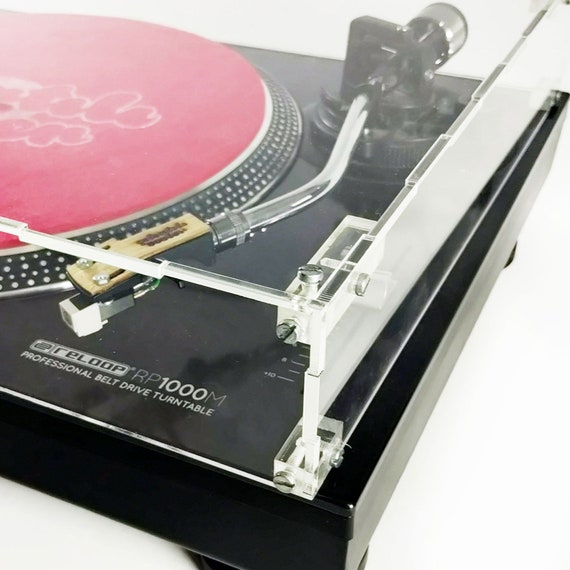In the color photograph, we see approximately three-fourths of a Reloop RP-1000M Professional Belt Drive Turntable. The turntable is angled at about 45 degrees, rotated clockwise, with visibility of the lower right and upper right corners. The black base of the turntable is partially encased in a white plexiglass top, which is in a closed position. The label on the lower right corner of the device reads "Reloop RP-1000M Professional Belt Drive Turntable," with "Reloop" enclosed in a white or gray box with black text, and the remaining text below it in a smaller font. 

The arm of the turntable extends outwards with a black base transitioning to a chrome finish, culminating in the needle. Adjacent to the arm on the left is a round circular metal base featuring small dots. On top of this base, there is a flat red surface adorned with a scroll-like cloud design in the center, suggesting either a decorative element or a felt cloth. Notably, the turntable is not currently in use, as there is no record present, and the needle is positioned to the left, away from the playing area.